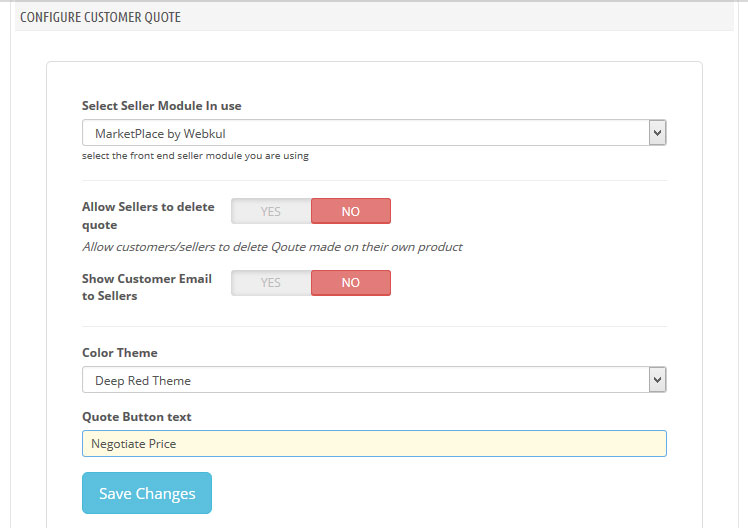The image depicts a user interface for configuring customer quotes on a web platform. At the top, there's a prominent gray box labeled "Configure Customer Quote" that spans across the interface. Below it, a white box contains several dropdown menus and options. 

The first section within this white box is titled "Select Seller Module." It includes a dropdown menu where users can choose from various seller modules. Another box beneath this section reads "Web Place" by "Web Cull."

Further down, the interface provides the option to "Allow Sellers to Delete Quote," accompanied by a yes/no toggle. The "No" option is highlighted in red. There's also an option that reads "Show Customer Email to Sellers," with another yes/no toggle where the "No" option is again highlighted in red.

Next, there's a "Color Theme" dropdown box for users to select the desired color scheme for the interface. Following that is a text input labeled "Quote Button Text," which contains the text "Negotiate Price" in a tan-colored box.

At the bottom of the interface, a blue box is labeled "Save Changes," allowing users to apply their configurations.

The image is primarily in black and white, making it straightforward and easy to understand, despite the accents of red, tan, and blue for specific interactive elements. There are no identifying logos or contact information visible in the image to indicate the owner of the website.